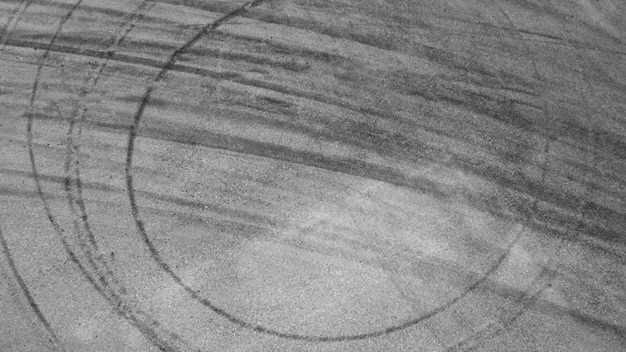This is a detailed black-and-white photograph, possibly of a pencil drawing, showing a complex design that features numerous concentric circles. The image has a translucent quality, hinting at some indistinct elements behind the main drawing. The circles are varied in their shading, with the first being the darkest and subsequent ones lighter. The scene may resemble a high-altitude view of a desert surface or runway, characterized by flat, gray tones. Prominent streaks of black lines cut horizontally across the circles, creating an impression of movement similar to tire marks left by cars possibly doing donuts. Gray rectangular shapes with intricate lines and circles are interspersed throughout, adding a unique, abstract layer to the overall composition. The photograph's gray table-like background supports the artwork, enhancing the visibility of the outlined circles and lines.